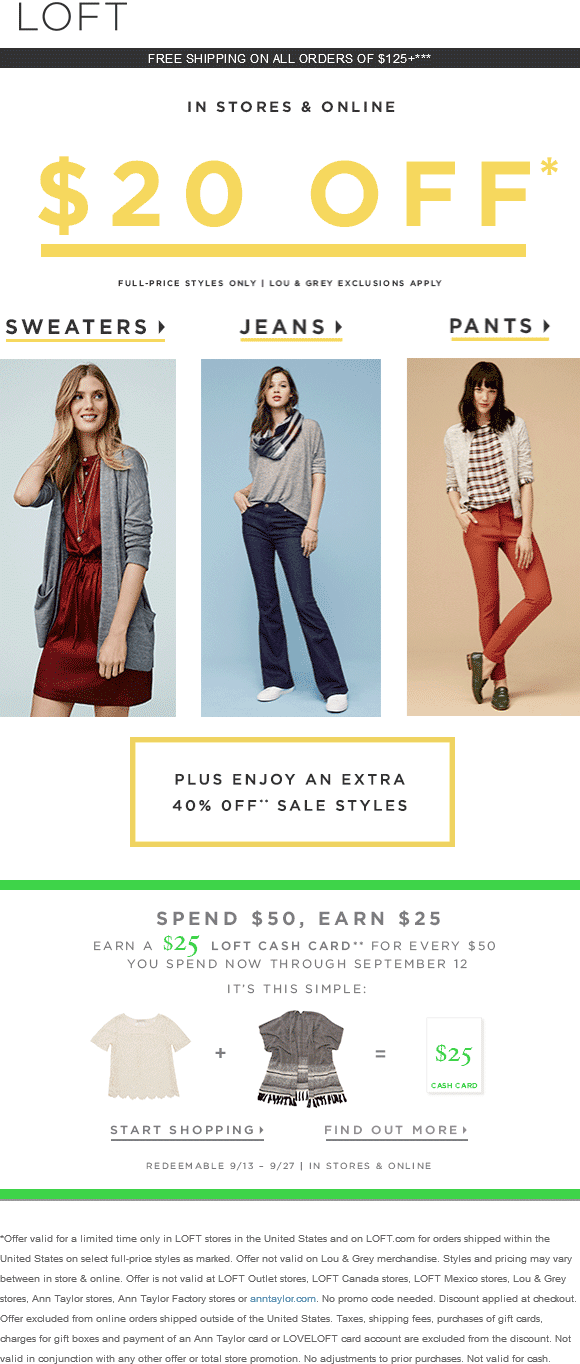**Loft Mobile Advertisement**

At the top of this vertically-oriented mobile advertisement, the Loft logo is prominently displayed in the top left corner. Just below the logo, a black banner announces, "Free Shipping on all orders of $125+," punctuated by three asterisks.

Underneath the banner, it states, "In stores and online," followed by a bold and large dollar sign accompanying the text "$20 Off." This section features additional details in smaller print, clarifying "Full price styles only, exclusions apply" in blue and grey text.

The visual layout is divided into three primary segments showcasing different apparel categories:

1. **Sweaters:** Featuring an image of a woman with blonde hair wearing a red dress paired with a grey sweater.
2. **Jeans:** Depicting a woman in blue jeans and a grey shirt adorned with a scarf, set against a blue background.
3. **Pants:** Highlighting a woman with black hair dressed in orange pants, a checked shirt, and a sweater.

Beneath these images, a boxed section announces, "Please enjoy an extra 30% off** sale styles," with a green line extending horizontally below it.

Further down, there's a promotional offer stating, "Spend $50, Earn $25." It details that for every $50 spent now through September 12th, customers will earn a $25 Loft Cash Card. The message includes a visual equation featuring a picture of a shirt, a plus sign, and a sweater, leading to the $25 cash card image. The section concludes with "Start shopping, find out more."

At the bottom, it specifies that the earned cash cards are redeemable from September 13th to 27th, applicable in stores and online. Another green line segments this part of the advertisement from additional information listed beneath it.